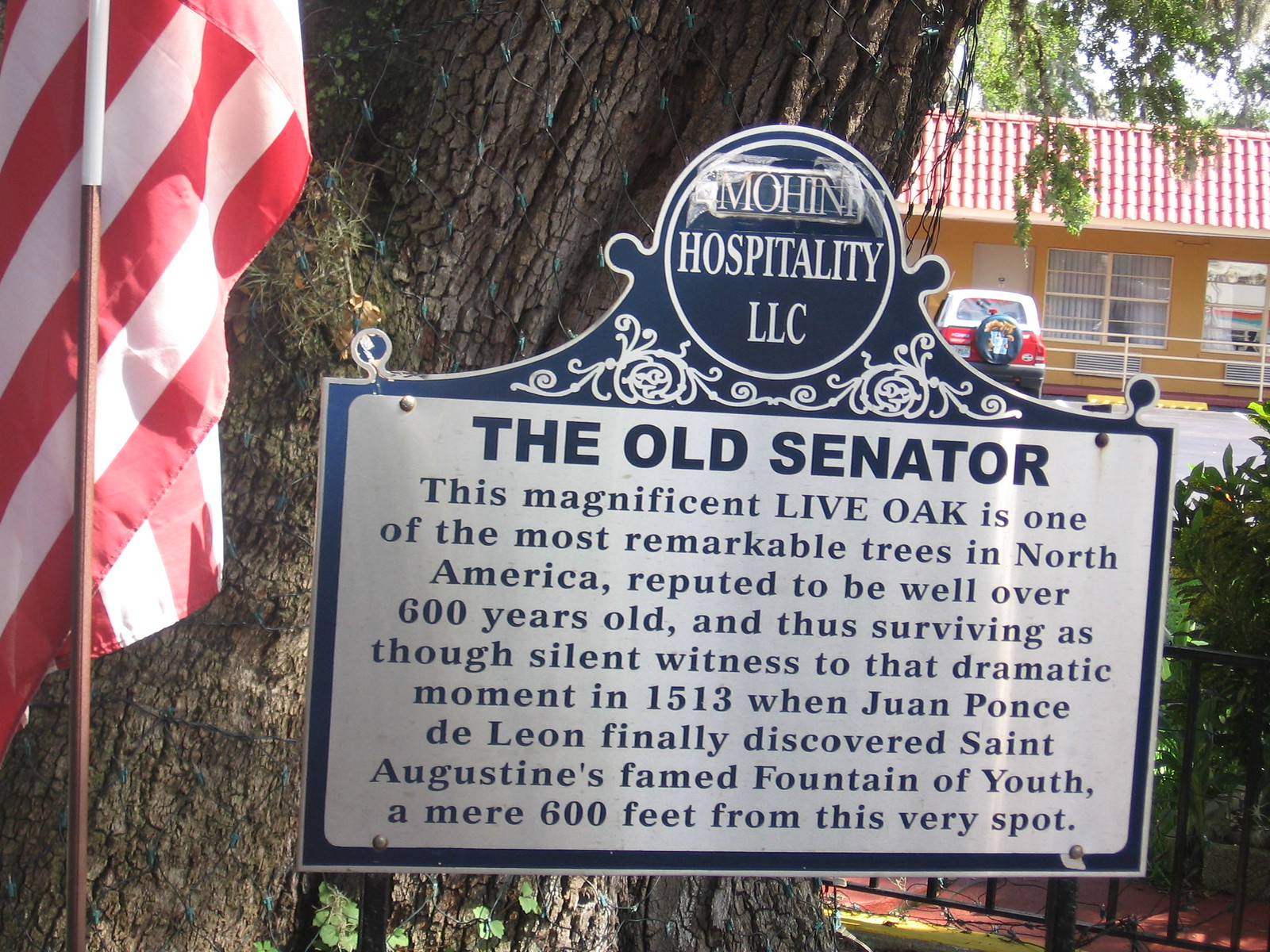The image features an outdoor scene centered around an ornate, metallic sign bolted to metal poles. The top of the sign is circular and reads "Mohini Hospitality LLC." Below, on a white background with black text, it describes "The Old Senator," a magnificent live oak tree believed to be over 600 years old. This tree is noted as one of North America's most remarkable oaks and a silent witness to Juan Ponce de Leon's 1513 discovery of St. Augustine's famed Fountain of Youth, just 600 feet away. Surrounding the sign and tree, several details enrich the scene: the trunk of the ancient oak is immense and wrapped in Christmas lights; an American flag is positioned to the left; and a yellow building, partially visible, sits in the background along with a parked car. The photo, taken during the daytime, showcases colors such as red, white, blue, gray, brown, yellow, green, and pink, and suggests the location might be near a restaurant or a famous historical site.